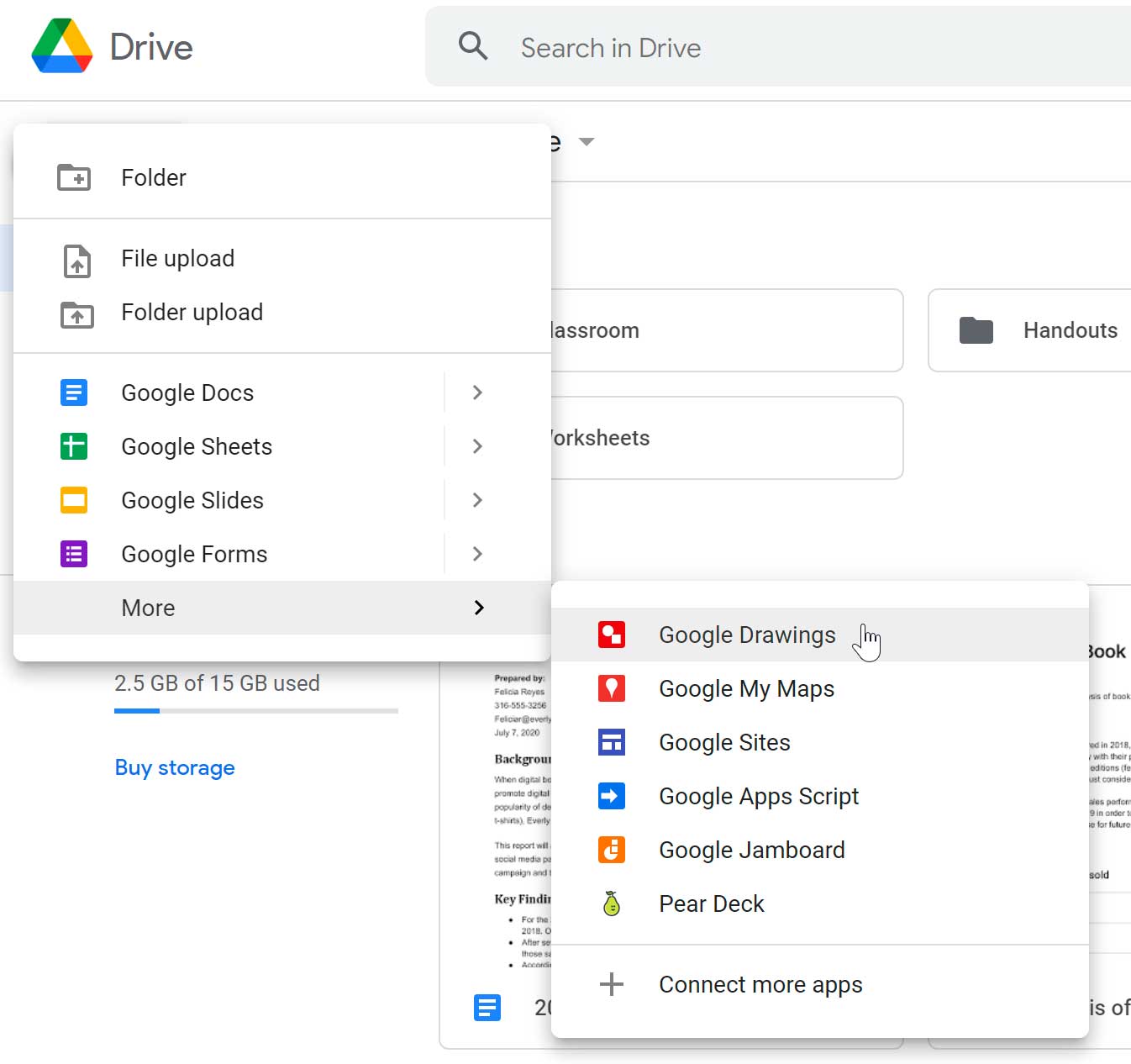The image is a screenshot of a Google Drive interface displayed within a web browser, characterized by its crisp white background. In the upper left-hand corner, the iconic Google Drive logo is prominently featured—a triangular ribbon design incorporating Google's signature colors: green, white, red, yellow, and blue. Adjacent to the logo is an elongated rectangular search bar bearing the placeholder text "Search in Drive."

The user has interacted with the interface, triggering a pop-up menu. This menu is a square-shaped prompt that provides a variety of options: the ability to create a new folder, upload files, upload folders, and access several Google productivity tools such as Google Docs, Google Sheets, Google Slides, and Google Forms. Each of these options is accompanied by a rightward-facing arrow, suggesting the availability of further sub-menu items.

At the bottom of this initial pop-up, there is a "More" option, also marked with a rightward-facing arrow. Selecting "More" has caused a secondary pop-up menu to appear, displaying additional Google applications including Google Drawings, Google My Maps, Google Sites, Google Apps Script, Google Jamboard, and Pear Deck. The screenshot captures these layered interactions in a comprehensive yet streamlined interface design.